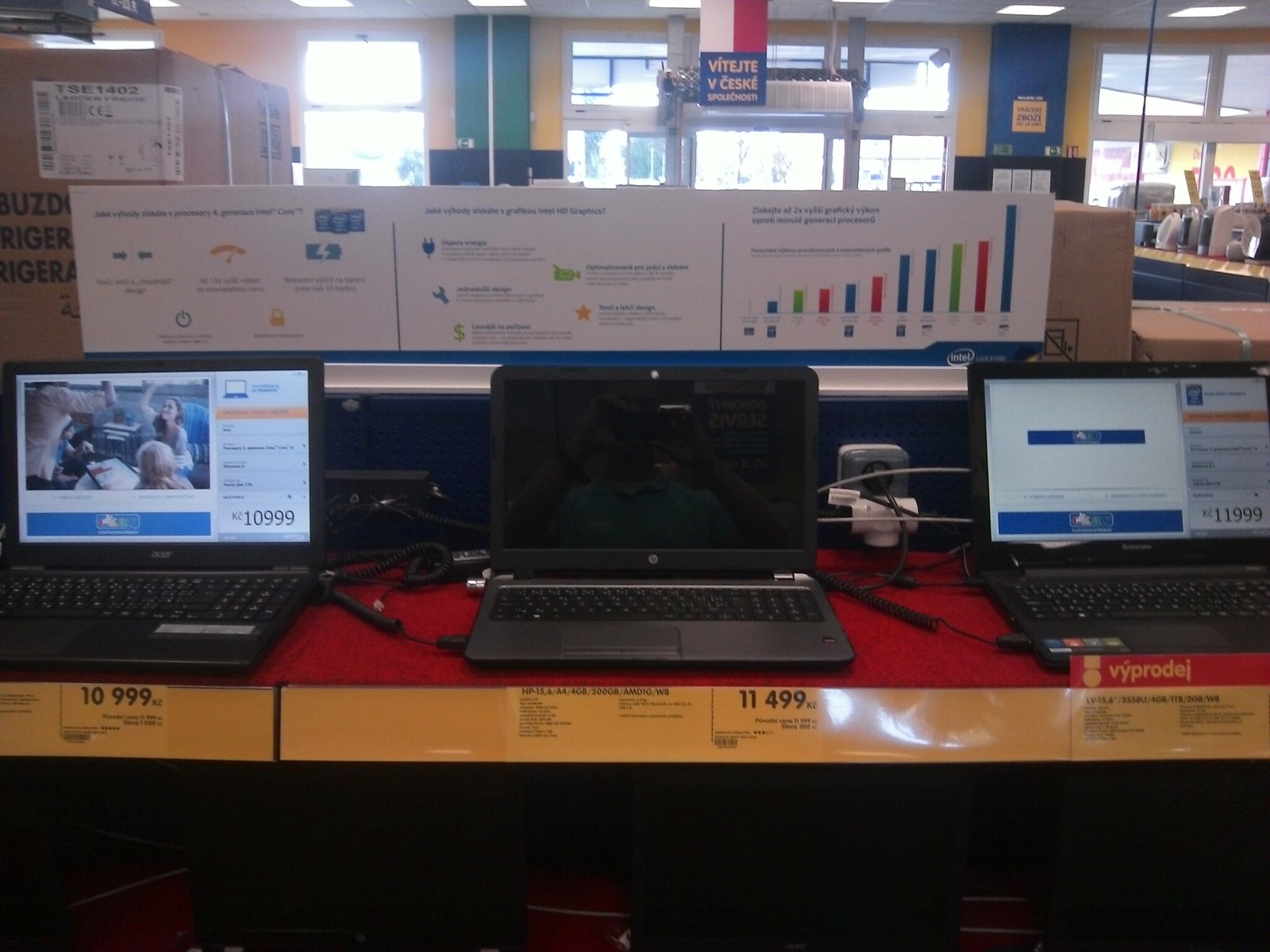This photograph captures a store display featuring three laptops prominently positioned on a display desk. The laptops on the outer ends are turned on, while the central laptop is turned off and displays a reflection of a person taking the photograph. The middle laptop, identified by the HP logo, is priced at $11,499, with its details and pricing indicated on a card beneath it. Similarly, the laptop on the left is priced at $10,999, with its details displayed below it. The right-side laptop, priced at $11,999, also has a card that is visible in the picture. The background reveals brightly lit surroundings, various shelves with electronic devices, colorful charts, and some cardboard boxes, suggesting a well-stocked and organized retail environment. Additionally, natural light floods the room through windows, further illuminating the display. The language on the labels suggests a European setting.